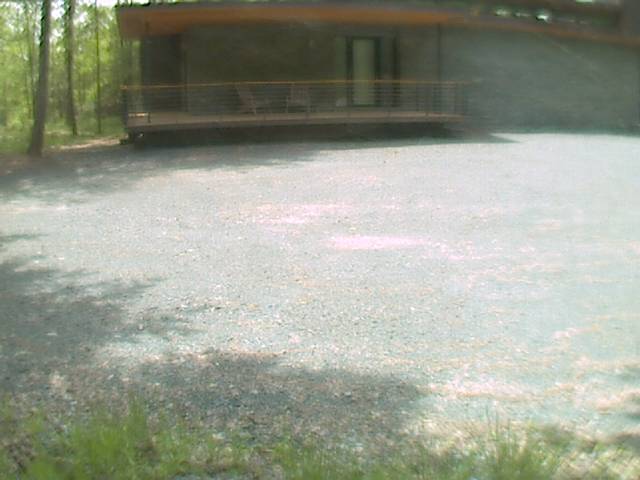This outdoor photograph, albeit blurry and possibly distorted by dust or dirt, features an isolated, contemporary guest house situated in a rural area, surrounded by a dense forest of tall trees. The house appears gray with a tan porch that extends partially around its front. A prominent white door with black trim can be seen, leading onto a small fenced-in deck with a railing that is roped off, possibly with yellow crime scene tape. Two Adirondack chairs are positioned on the porch, adding a quaint touch to the secluded scene. In front of the house lies a large gravel parking area, bordered by some overgrown grass and flanked by shadows of trees at the picture's edges.